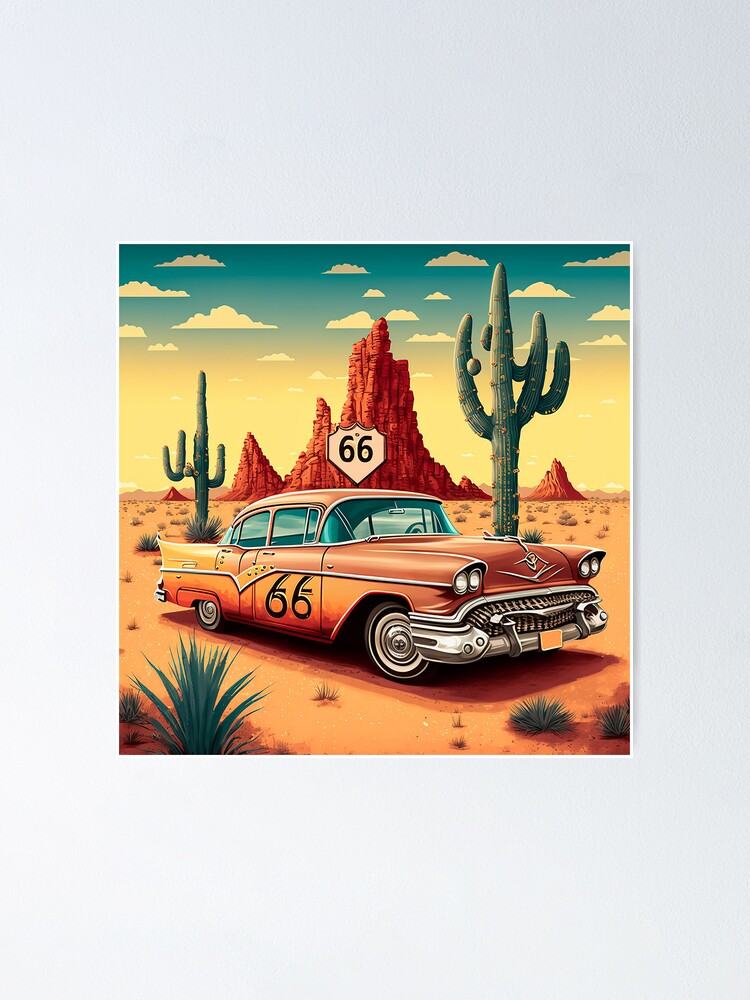This piece of digital art, hung on a canvas against a white wall, features an old-style car, reminiscent of a taxi cab, painted in a vibrant yellow-orange hue. The car, which sports a chrome grille and an emblem on its hood, is facing slightly to the right, allowing a view of both its front and right side. The number '66' is distinctly painted in black on the passenger door, indicating a connection to the famous Route 66. Behind the car, there's a prominent white sign also marked with '66' set amidst a desert landscape. Flanking the sign are cactuses, and spread across the scene are various small desert plants. In the background, sand dune-style mountains add depth to the scenery. The sky above transitions from yellow near the horizon to blue at the top, interspersed with white clouds.

The image is encased within a thick gray border, which is darker at the top and lighter at the bottom. The left and right sides of the border are relatively thinner. This border frames the colorful, animated square picture, enhancing its vibrant desert setting.